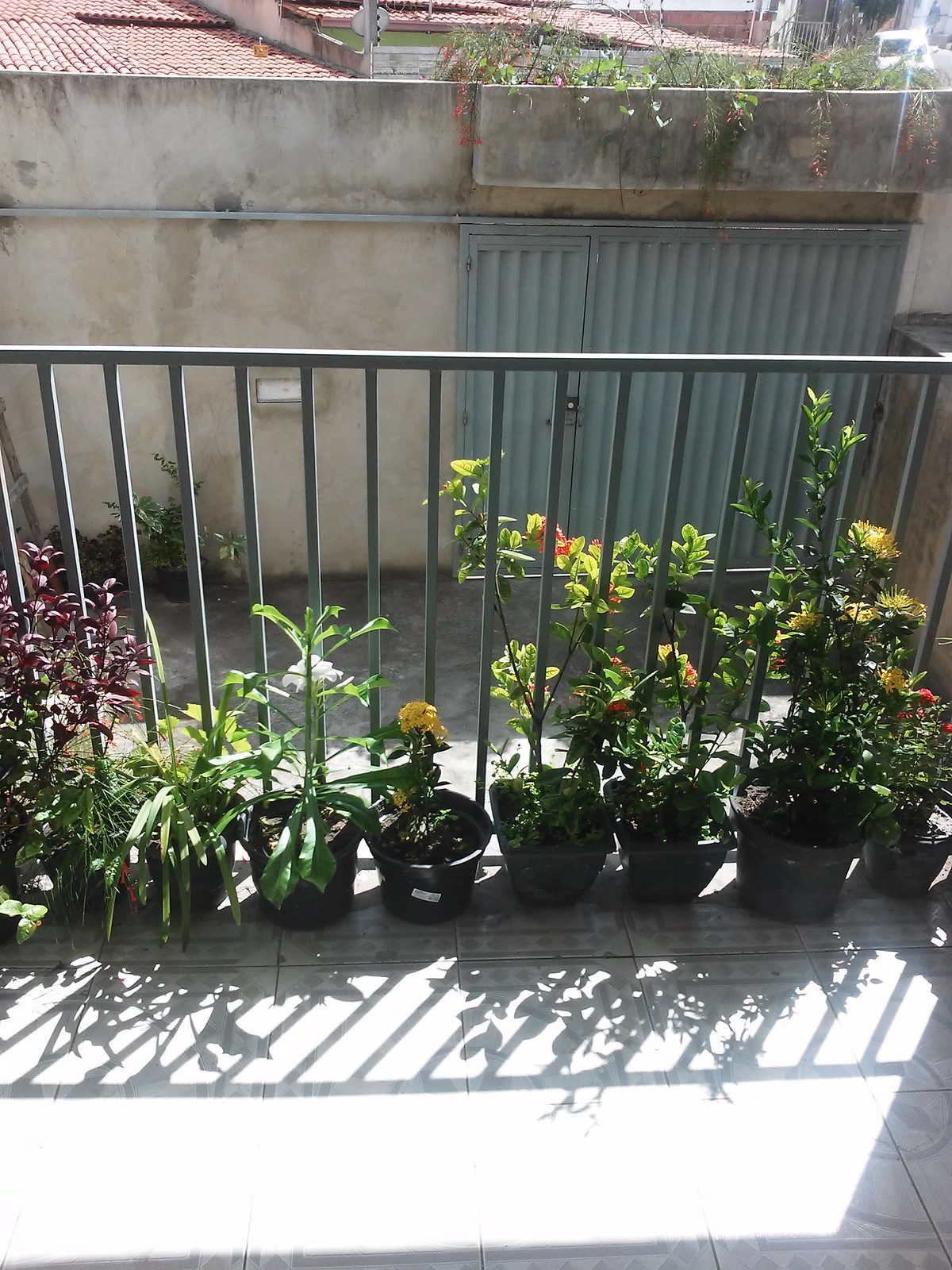This photograph, taken on a sunny day, captures a cozy balcony garden brimming with greenery and blooms. Positioned against a black metal railing, reminiscent of typical balcony guardrails, are eight distinct potted plants, each housed in dark containers aligned horizontally. The central plant showcases vibrant yellow flowers, while to its right, additional pots hold plants poised to blossom with more flowers, possibly white and yellow. To the left, the foliage transitions into bushier, leafy plants.

The balcony fencing, casting intricate shadows under the bright sunlight, frames the scene along with a faded, stained concrete wall at the back. A blue panel and a green, corrugated metal piece are visible on this weathered wall, adding a textured backdrop. Further right, a rose bush distinguishes itself with burgundy hues, and its shadow dances on the tile floor below.

Beyond this charming setup, rooftops of neighboring buildings peek into view, hinting at a higher vantage point, possibly a rooftop or an upper-level balcony. This serene snapshot not only showcases the diversity of the potted garden but also the intricate interplay of light and texture in the surroundings.